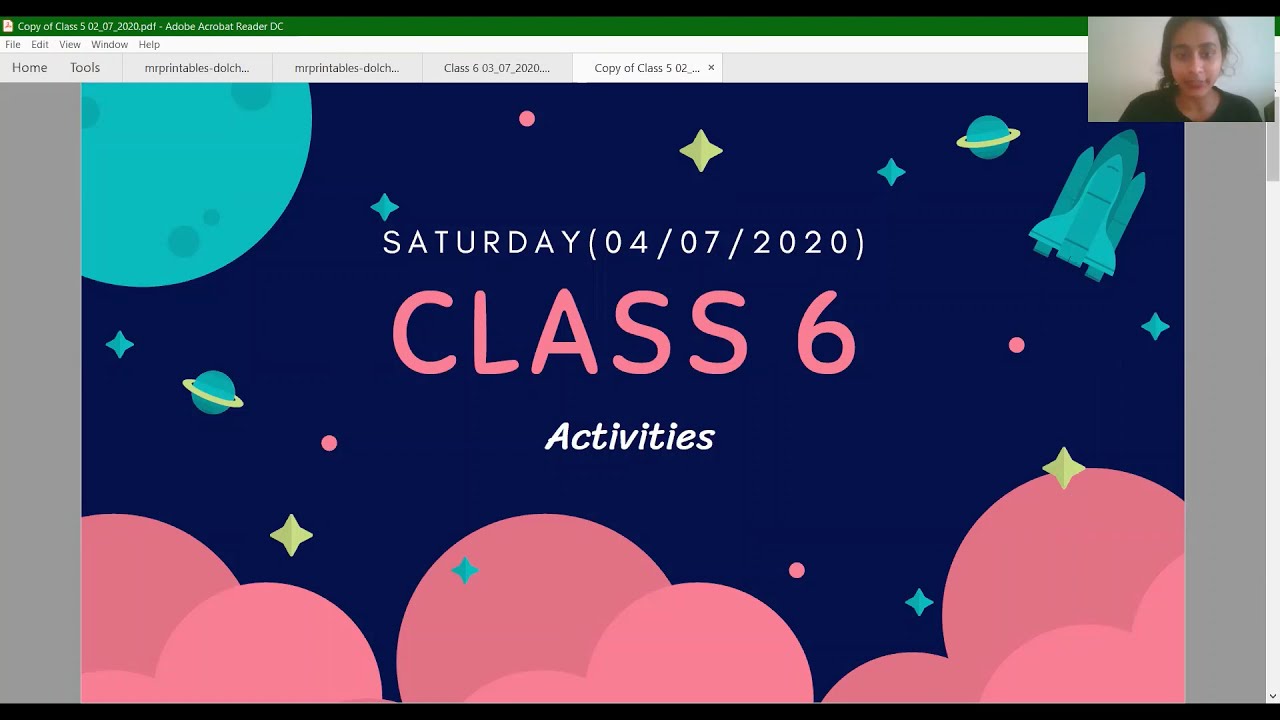This is a screenshot of a computer screen displaying a graphic design, likely part of a presentation or a background for a video communication platform. At the top of the screen, you can see a URL bar with multiple tabs, including ones labeled "home," "tools," and tabs associated with classes. The main content showcases a dark navy blue background adorned with a starry night theme. In the upper left corner is a round bluish planetoid, while overlapping pink circles embellish the bottom of the frame. A light blue space shuttle with a booster is stationed in the upper right corner, amidst various colored stars in teal, green, yellow, and pink.

The textual content is prominently displayed in the center. "Serve It Saturday" with the date "04/07/2020" is written in small block letters at the top. Below that, "CLASS 6" is boldly highlighted in large pinkish letters, with "Activities" in smaller, italicized cursive beneath it. In the upper right corner of the screen, there is a small video feed showing a woman, possibly South Asian or Indian, who appears to be the presenter or teacher. She has dark hair and is wearing a dark top. The overall design serves as an engaging and vibrant visual aid for what seems to be an online class session.